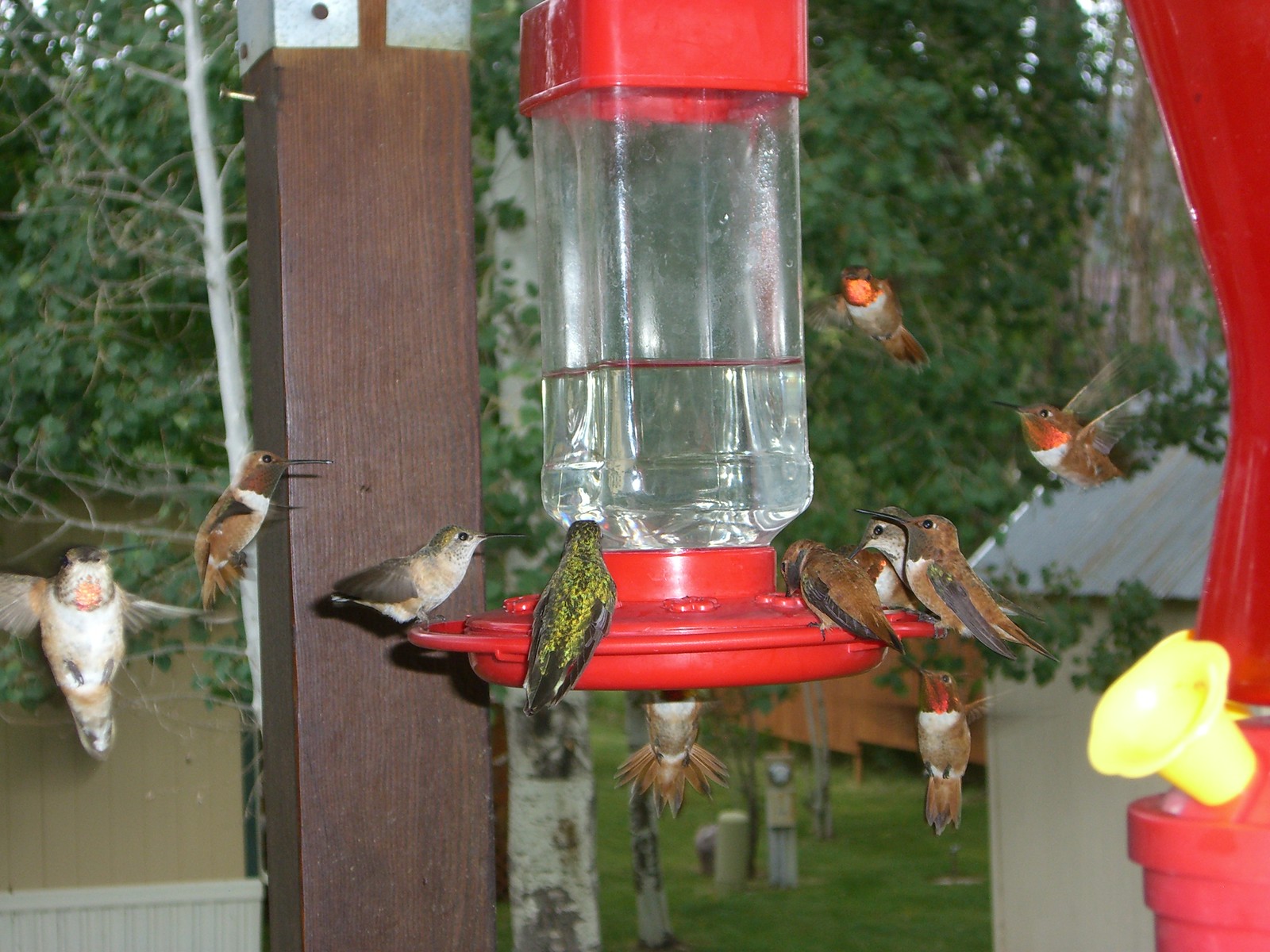An outdoor photograph captures a typical hummingbird feeder prominently in the center, hanging from what appears to be a back porch. This feeder features a red base and a red square cap, with a clear, rectangular prism-shaped glass body filled halfway with clear liquid. Due to the cropping of the picture, the very top of the feeder isn't visible. Perched on the feeder are about five or six hummingbirds, while another 12 to 14 birds hover mid-flight around it. The hummingbirds exhibit a variety of colors, including brown and white, green and white, and white and gray. The backdrop reveals a densely wooded area with abundant greenery, and a wooden post likely supporting the porch structure is visible to the left of the feeder. To the right, another hummingbird feeder peeks into the frame, partially cropped out.